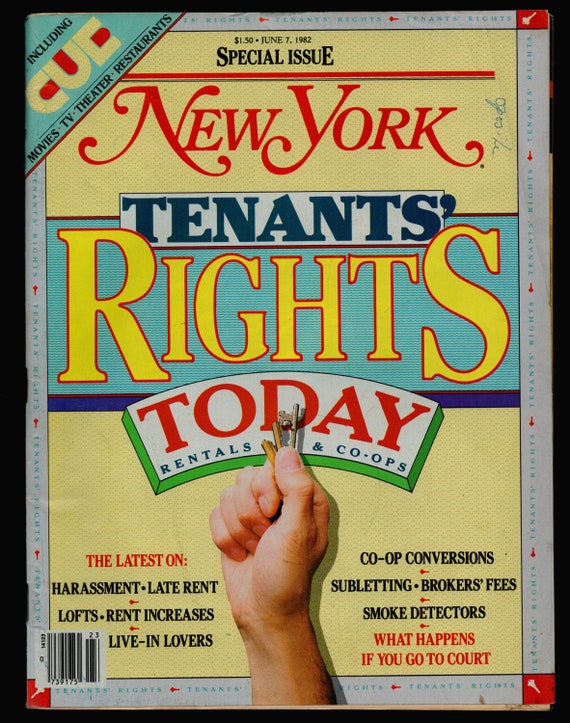This image is the cover of a special issue of New York magazine, dated June 7th, 1982, priced at $1.50. The background is predominantly yellow, framed by a light gray-blue border with red corners, and outlined in white. At the top left corner, a diagonal light blue section reads "including" in small black text, followed by "CUE" in large yellow font, and "Movies, TV, Theater, Restaurants" in smaller black text.

Central to the cover, in ornate red cursive, is the magazine's title, "New York." Beneath that, in bold black letters, it announces "Tenants," followed by "Rights" in prominent yellow font within a light blue rectangle, and "Today" in large red letters on a white arc. The lower portion of the cover features a Caucasian person’s hand, fist clenched, holding a set of keys. This central image partially obscures the word "Today."

The bottom of the cover furnishes a detailed overview of the issue's content in various colored fonts. It includes sections on harassment, late rent, lofts, rent increases, live-in lovers, co-op conversions, subletting, broker's fees, smoke detectors, and court proceedings, all addressed under the theme of tenant rights in rentals and co-ops.